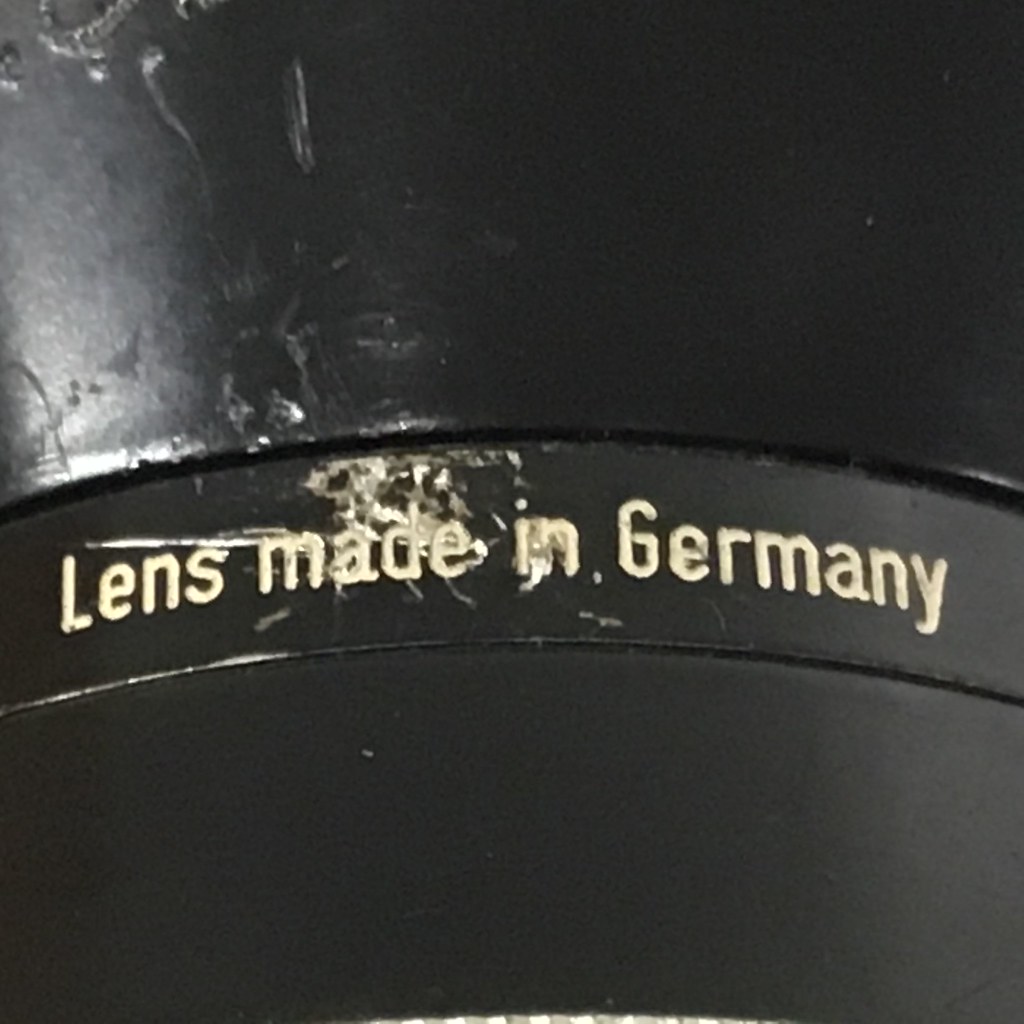This is an up-close, highly detailed photograph of a black camera lens, likely made of metal or plastic, that has seen better days. The surface of the lens is marred by numerous cracks and small scratches, predominantly concentrated in the center and extending to the top left. Engraved prominently in the middle is the white text, "lens made in Germany," framed by two small indentations that border the text. The lower part of the lens appears less damaged in contrast to the extensively scratched upper areas. Light is reflecting off the left side, enhancing the shiny black appearance of the less damaged metals. The multitude of scratches and potential burn marks suggests the lens has had a rough history, reflecting a story of heavy usage and perhaps neglect.